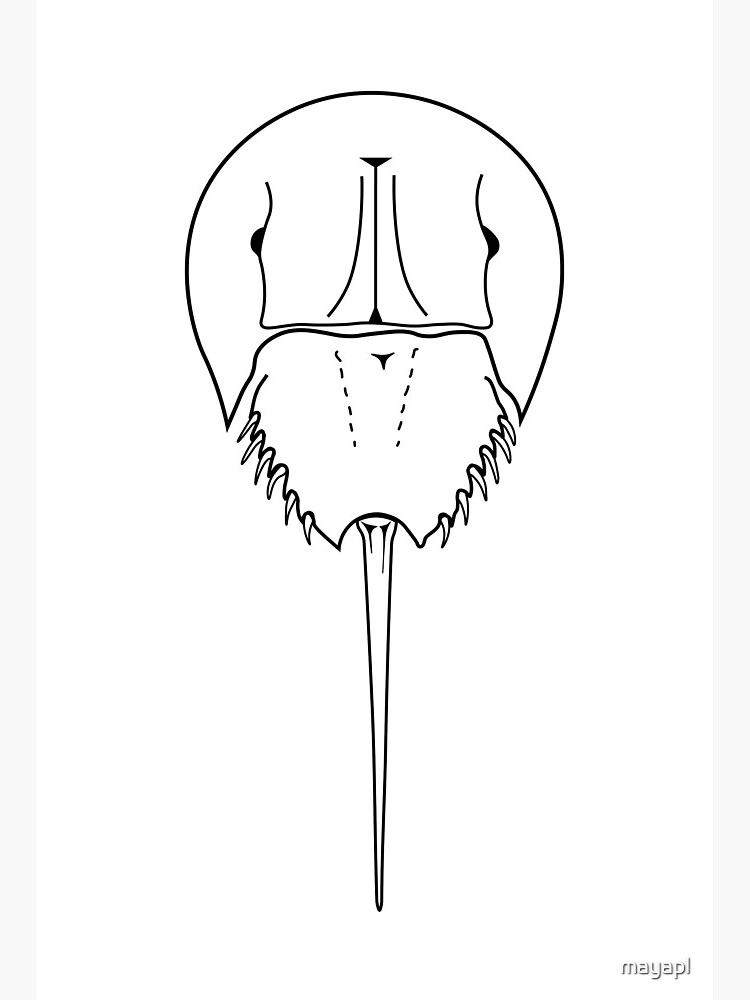The image depicts a highly detailed, black and white digital drawing of a horseshoe crab positioned at the center of the composition. The background is stark white, with thin, light gray lines framing the left and right edges, giving the appearance of an art print. The horseshoe crab is oriented with its head towards the top and its tail extending downwards. The body of the crab is divided into two main sections: the front, which resembles a half-circle with a slightly pear-shaped top, and the rear, which features a long, sharply pointed, elongated tail. The shell shows intricate details, including wavy lines and black dots indicating the eyes on either side of a central line that runs from the head to the tail. The lower part of the shell is adorned with black striped lines. At the bottom right corner of the image, the text "Maya PL" is displayed in all lowercase letters, bordered by a thin black outline.